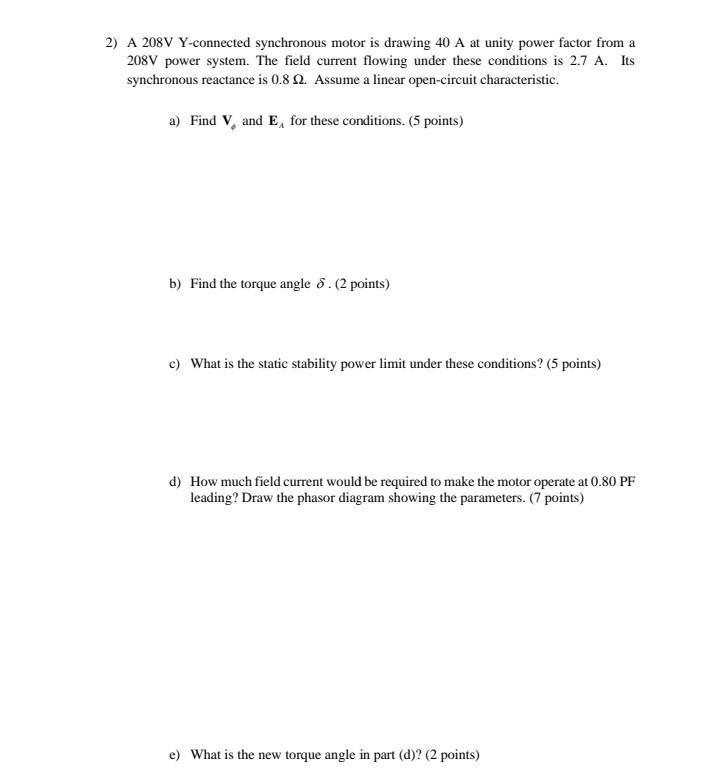The image shows a portion of an exam or quiz from what appears to be a college-level course, likely in physics or electrical engineering. The specific question is number 2 and reads: "A 208V Y-connected synchronous motor is drawing 40A at unity power factor from a 208V power system. The field current flowing under these conditions is 2.7A, and its synchronous reactance is 0.8Ω. Assume a linear open circuit characteristic." There are subsections labeled A through E, each associated with a specific point value, such as Part A worth 5 points, aimed at finding V and E under these conditions; Part B worth 2 points to find the torque angle, and others that include inquiries on static stability power limit. The question and sub-questions are presented in black text on a white background, adhering to a format typical of a structured exam or textbook.